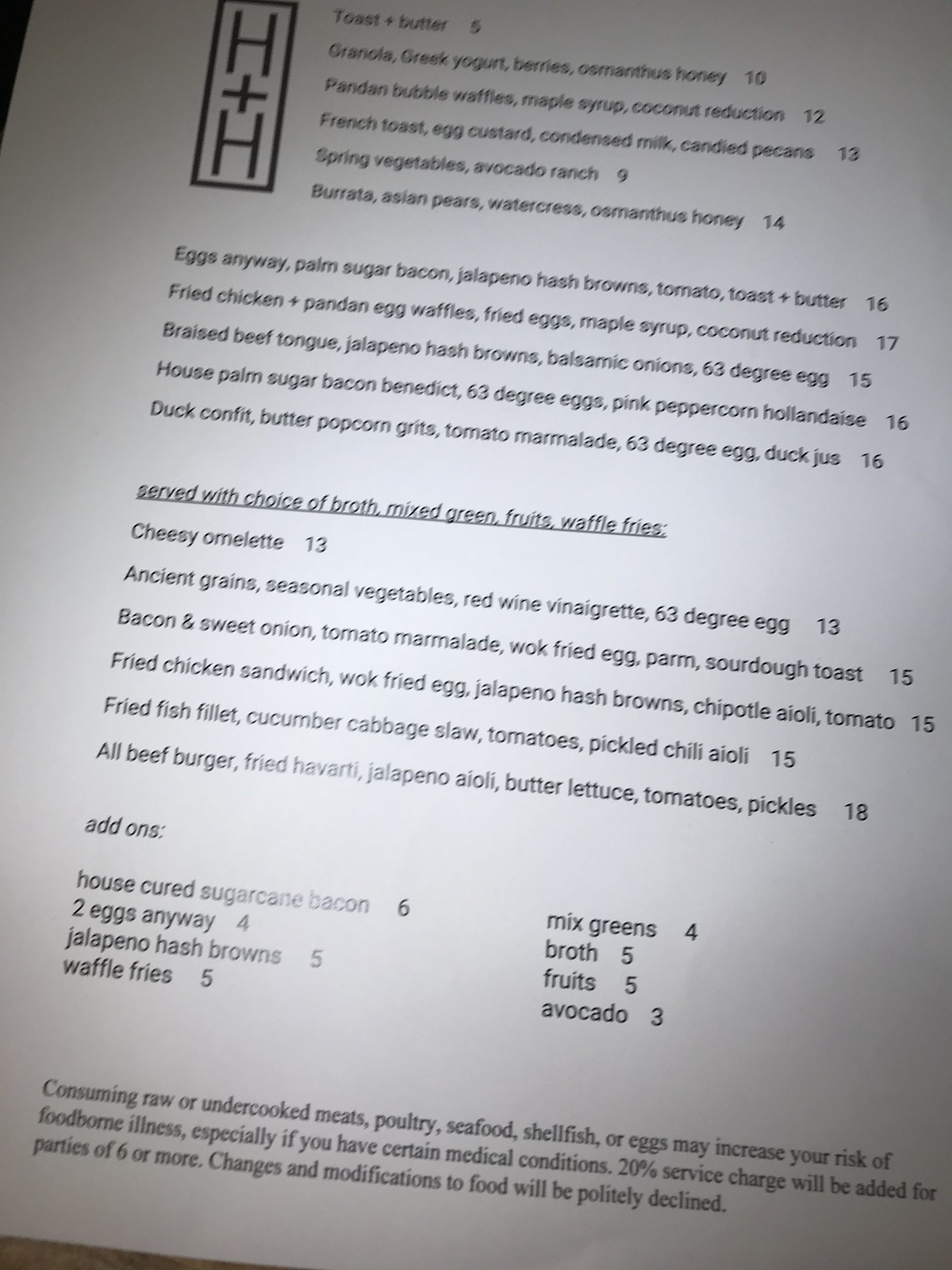This is an image of a restaurant menu displayed against a plain white background. In the upper left corner, there is a distinctive black box containing a black letter "H." The menu text, primarily black, is organized into several rows and sections, although the top portion is slightly cut off at an angle, giving a slanted view of the text.

The menu items are listed as follows:
1. **Coconut Reduction** - $12
2. **French Toast**: Egg custard, condensed milk, candied pecans - $13
3. **Spring Vegetables**: Avocado, ranch - $9
4. **Burrata**: Asian pears, watercress, atha, manthas, honey - $14

There is a noticeable break in the text before the following items:
5. **Eggs Any Way**: Palm sugar bacon, jalapeno hash browns, tomato toast and butter - $16
6. **Fried Chicken + Pandan Egg Waffles**: Fried eggs, maple syrup, coconut reduction - $17
7. **Braised Beef Tongue**: Jalapeno hash browns, balsamic onions, 63-degree eggs - $15
8. **House Palm Sugar Bacon Benedict**: 63-degree eggs, pink peppercorn hollandaise - $16
9. **Duck Confit**: Butter popcorn grits, tomato marmalade, 63-degree eggs, duck jus - $16

Below this, there's a section with underlined text indicating that dishes are served with a choice of broth, mixed greens, fruits, and waffles. Additional items are listed below:
- **Cheesy Omelet**
- **Ancient Grains**
- **Seasonal Vegetables**
- **Red Vinaigrette**

This runs for a couple more lines before breaking into the add-ons section, which is divided into two columns. Add-ons include various meats, eggs, hash browns, fries, fruits, broths, avocados, and mixed greens, each with its price.

At the very bottom of the menu, there's a disclaimer regarding the consumption of raw or undercooked meats.